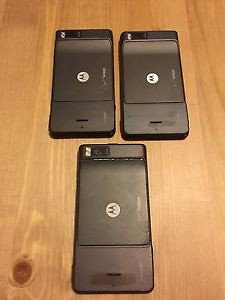This color photograph captures a close-up of three matte-black Motorola smartphones, likely from the mid-90s to early 2000s, arranged on a natural, light pine-colored wooden table. The table's grain runs vertically with a prominent dark brown knot on the bottom left. The phones are laid face down, showing their back panels which feature a white Motorola emblem, a circle with a stylized "M". Each phone has a camera lens and flash in the upper left corner and a small rectangular groove at the bottom, possibly for battery removal. The consistent lighting highlights the light tan lines running through the table, adding texture to the scene. The photo is sharply focused, clearly revealing the used state of the devices and their specific design elements.